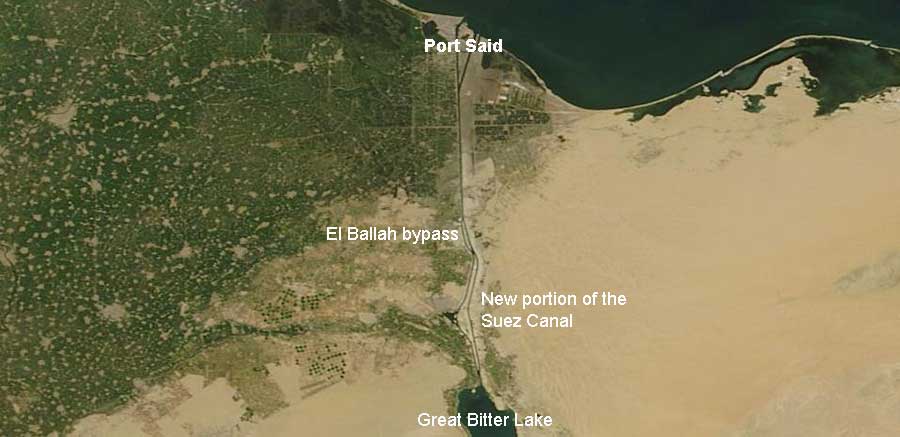This is an aerial image resembling a map, possibly taken from a high altitude, showing a detailed layout with prominent geographic and infrastructural features. At the top of the image, “Port Said” is labeled, hinting at the proximity to a large body of water visible in the top center and right, likely an ocean or expansive sea, partially cut off by the image's edge. The image is divided by a road labeled “El Bala Bypass” running vertically. To the left of this road, the area is predominantly green with patches of brown, suggesting vegetation interspersed with open lands. The left side also contains a small body of water labeled “Great Bitter Lake” near the bottom center. To the right of the El Bala Bypass, the area transitions to a predominantly brown, desolate, desert-like terrain with sparse greenery. This side features the “New Portion of the Suez Canal,” tracing a path from the road downwards and converging with the Great Bitter Lake. The labels on the image are in white, making them stand out clearly against the varied background, aiding in identifying the significant landmarks and geographical features.